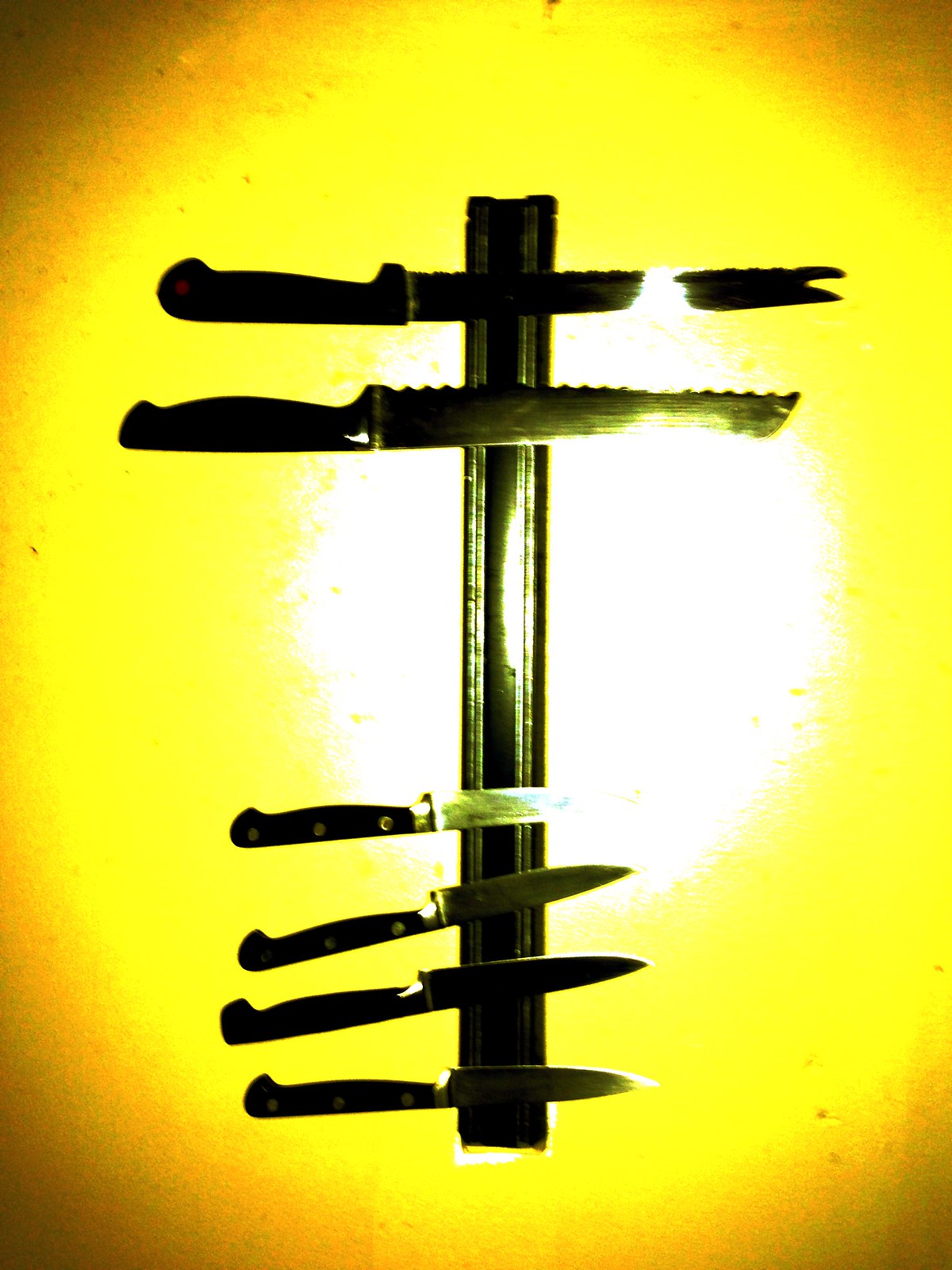The image features a vertical magnetic knife holder set against an intricate and vibrant yellow-toned background. The backdrop showcases a dramatic gradient that starts with a bright white circle at its center, gradually transitioning to a fluorescent yellow, then to a darker yellow, and finally to tan in the corners, resembling a sunburst or light effect. The background might either be a painted surface or influenced by lighting, creating a glowing, almost diffused appearance. Mounted on the magnetic strip are six knives: two longer ones at the top with black handles—the first featuring a smooth blade and the second a serrated edge—and four smaller knives at the bottom, likely three steak knives and a paring knife, all silver-bladed with black handles. The image captures the knives horizontally aligned on the vertical magnetic strip, creating a symmetrical and balanced arrangement, giving the entire setup an artistic yet practical look.